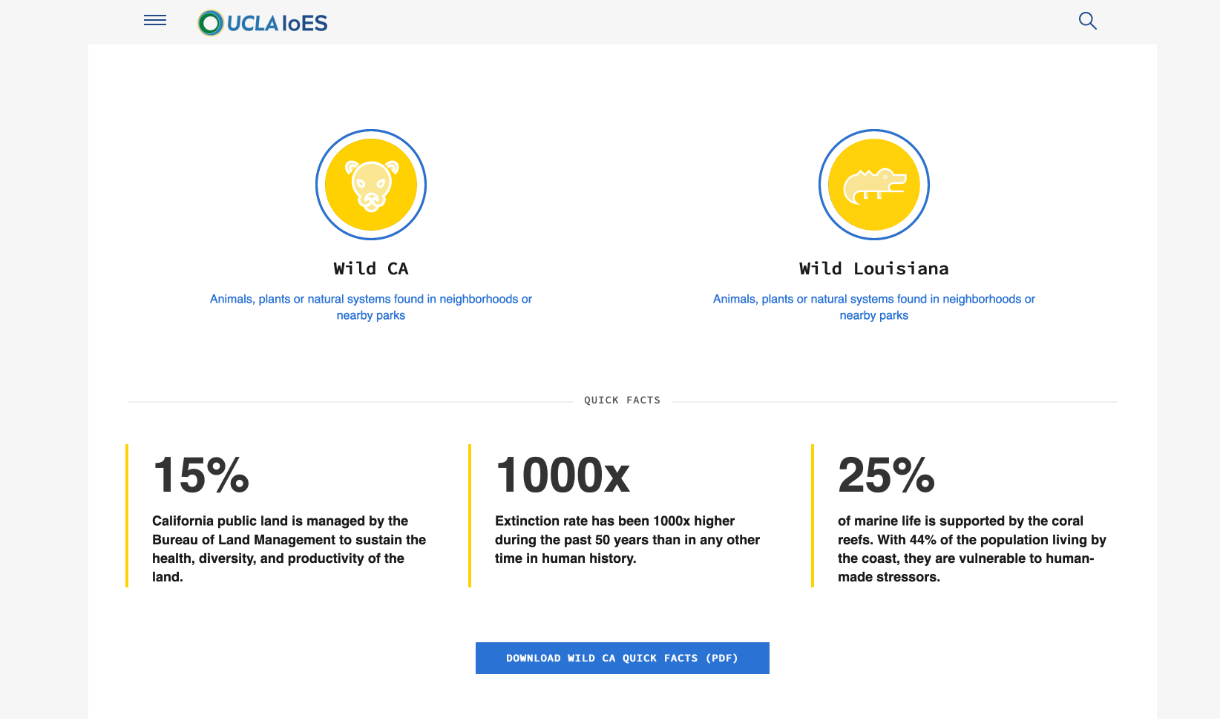#### Detailed Caption for the Screenshot Image:

The screenshot features a light gray background with a navigational bar at the top. Approximately 20 spaces from the left margin, there is a blue hamburger menu icon. Adjacent to this icon is a green outlined circle. To the right of this, the text "UCLA" is displayed in light blue, followed by "LOES" in darker blue. On the far right of the top bar, there is a blue magnifying glass icon.

The main portion of the screen is occupied by a large white square. At the top corners of this square are two yellow circles outlined with a thin blue line. The left circle contains a white bear head, and below it, in bolded black text, is "Wild CA." Underneath, in blue text, the following description is provided: "Animals, plants, or natural systems found in neighborhoods or nearby parks."

The right yellow circle contains the image of an alligator. Below this circle, in bolded black text, is "Wild Louisiana," followed by the same blue text description as the left side.

About five lines down, a light gray horizontal line spans the width of the white square. Centered on this line, in small gray letters, is the phrase "Quick Facts."

Below this section, the content is organized into three columns separated by vertical yellow lines:
- The left column features a bolded "15%" sign. Below this, the text reads: "California public land is managed by the Bureau of Land Management to sustain the health, diversity, and productivity of the land."
- The center column is headed by a bold "1000X," followed by: "Extinction rate has been 1000X higher during the past 50 years than in any other time in human history."
- The right column states: "25% of marine life is supported by coral reefs. With 44% of the population living by the coast, they are vulnerable to human-made stressors."

At the bottom of the screen, a blue rectangular button with white text inside reads: "DOWNLOAD WILD CA QUICK FACTS (PDF)."